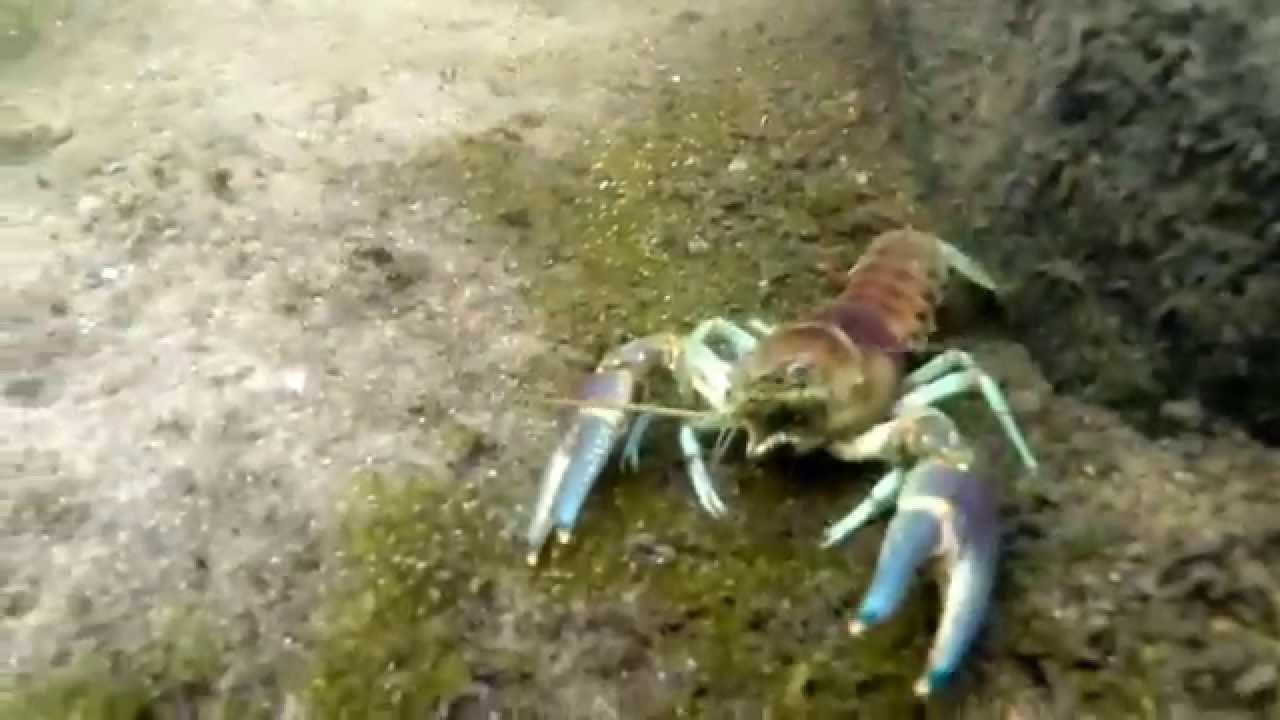The photograph captures an underwater scene featuring a unique crustacean that appears to be a hybrid of a lobster and a crab. The crustacean, positioned at the bottom of the ocean, is surrounded by debris and algae-covered sand, with a large black rock behind it. The animal itself is striking in coloration: its main body is a dark reddish-purple, almost fluorescent in appearance, while its claws are a vivid blue with hints of purple, and its legs are light green. The crustacean's claws are open and it seems to be facing towards the camera. The image quality is low and somewhat blurry, reminiscent of footage from older underwater cameras, which could explain the somewhat altered colors and pixelation. The presence of sand, algae, and a big rocky area adds context to the underwater habitat.